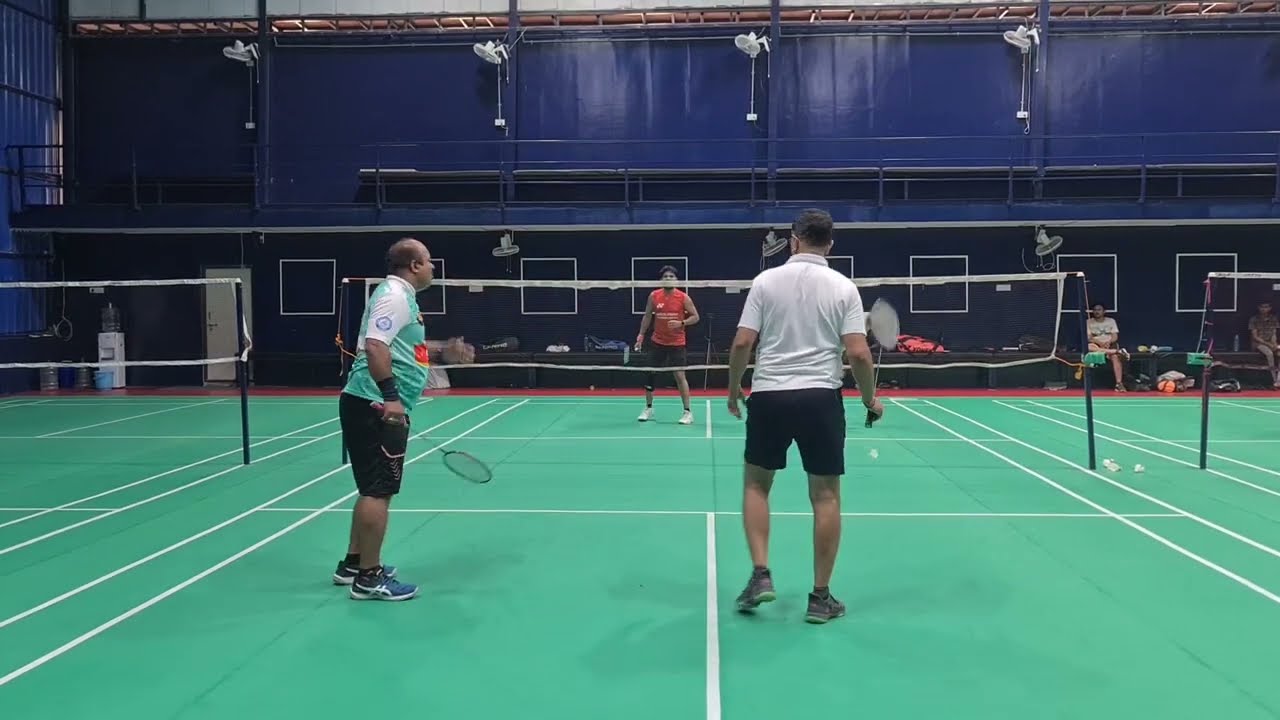In this detailed indoor scene, we see an intense badminton match unfolding on a lime green court with crisp white lines. The court, located in a building with dark blue walls that extend up to a two-story height, is flanked by a center net dividing the playing area. On the left side of the court stands a bald man wearing a green and white short-sleeved jersey, black shorts, and blue tennis shoes, holding a racket in his right hand while his left hand is poised in front of his body. Next to him, slightly to the right, is a taller man with brown hair, dressed in a white, collared polo shirt, black shorts, and dark purple tennis shoes, also wielding a racket in his right hand. On the opposite side of the net is a man in a red sleeveless shirt, black shorts, and white tennis shoes. He appears focused, possibly preparing to return an incoming shot. He also seems to be wearing a knee brace on his right leg and has black socks on. The building's features include a row of benches along the side wall, with a couple of people seated on the far right-hand side, a water jug, a white door, and windows designed for safe viewing of the game. Overhead, multiple fans hang from the ceiling, ensuring the court remains cool, and a walkway up top is lined with bright lights, ready to illuminate the scene.